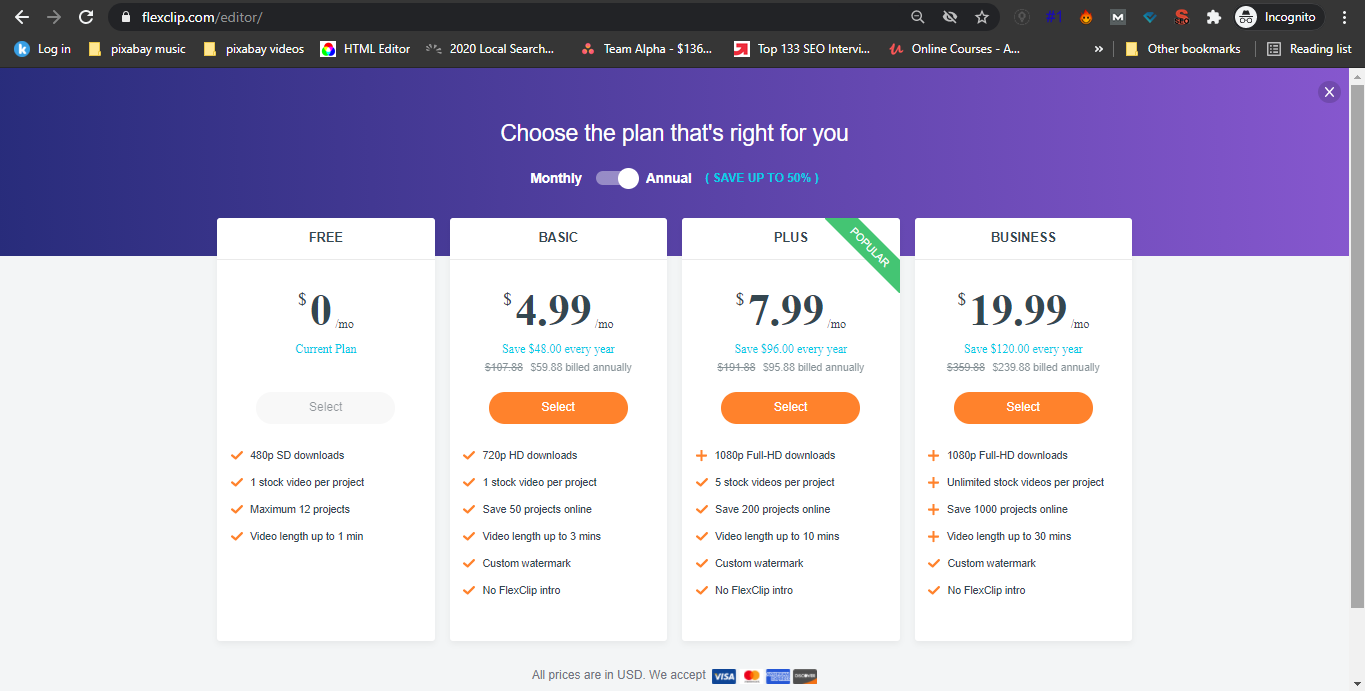This image is a detailed screenshot of a computer webpage, displaying a subscription plan comparison on the FlexClip website, specifically found at flexclip.com/editor. The top of the webpage features a purple background, with white text that reads, "Use the plan that's right for you." Users are presented with the option to choose between monthly and annual billing cycles, with a highlighted note indicating potential savings of up to 50%.

The subscription plans are organized into four tiers:

1. **Free Plan**:
   - Price: $0/month
   - Features:
     - 480p standard definition downloads
     - 1 stock video per project
     - Maximum of 12 projects
     - Video length up to 1 minute

2. **Basic Plan**:
   - Price: $4.99/month
   - Annual Savings: $48/year if billed annually
   - Features:
     - 720p HD downloads
     - 1 stock video per project
     - Save up to 50 projects online
     - Video length up to 3 minutes
     - Custom watermark
     - No FlexClip intro

3. **Plus Plan** (Most Popular):
   - Price: $7.99/month
   - Annual Savings: $96/year if billed annually
   - Features:
     - 1080p full HD downloads
     - 5 stock videos per project
     - Save up to 200 projects online
     - Video length up to 10 minutes
     - Custom watermark
     - No FlexClip intro

4. **Business Plan**:
   - Price: $19.99/month
   - Annual Savings: $120/year if billed annually
   - Features:
     - 1080p HD downloads
     - Unlimited stock videos per project
     - Save up to 1,000 projects online
     - Video length up to 30 minutes
     - Custom watermark
     - No FlexClip intro

At the bottom of the screenshot, a note specifies that all prices are in USD and lists the credit cards accepted for payment.